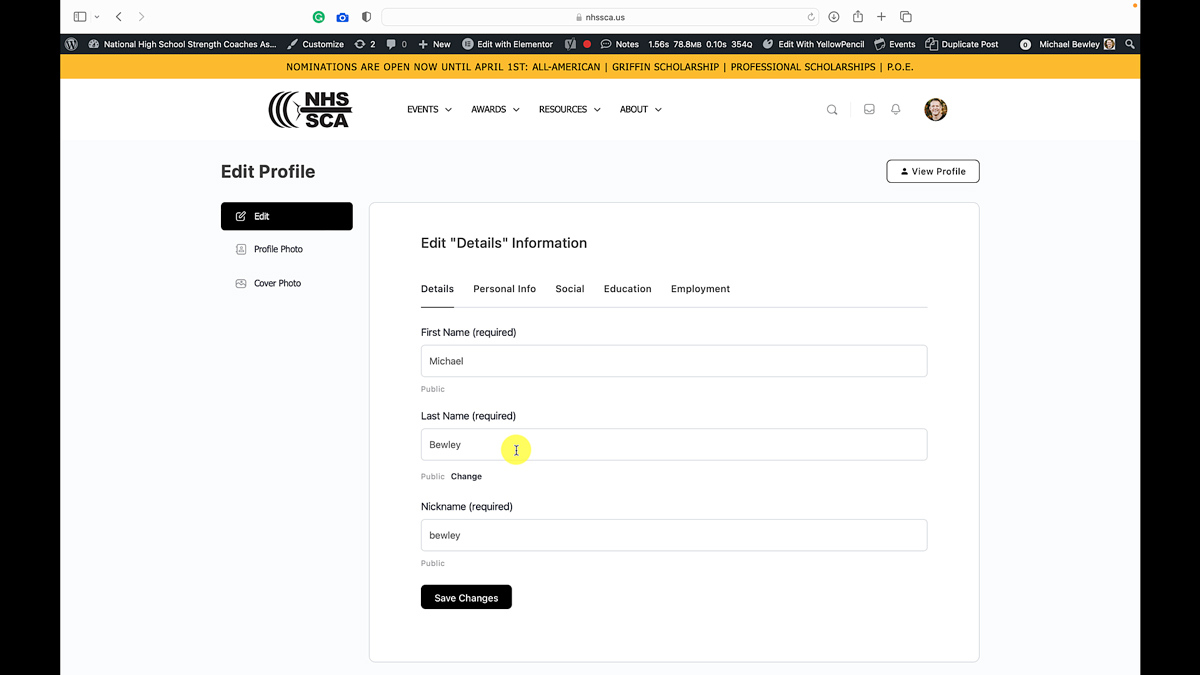This is a screenshot from a desktop web page for the National High School Coaches Association (NHSCA) profile section. At the very top, there is a white navigation bar featuring various icons on the left side, with the text "NHSCA.us." On the right side, there are additional icons. Below the navigation bar, there's a black bar with several truncated options, making it somewhat difficult to read. It mentions "High School Strength Coaches" and includes options such as "Customize," "New," "Edit with Elementor," "Notes," a phone number, "Edit with View Pencil," "Yellow Pencil," "Events," "Duplicate Post," and "Michael Burlap" with an associated profile picture icon.

Beneath the black bar, there's an orange banner announcing that nominations are open until April 1st for various programs including All-American, Griffin Scholarship, Professional Scholarships, and POE. The text "NHSCA" appears below this banner, accompanied by an icon resembling three crescent moons on the left. The subsequent navigation items in black text include "Events," "Awards," "Resources," and "About," each with dropdown menus. Additionally, there are icons for a magnifying glass (search), an envelope (messages), and a bell (notifications), followed by a profile picture likely representing Michael Burlap.

The main profile section below these navigation elements features a box labeled "View Profile" on the left side, alongside options to "Edit Profile," "Edit Profile Photo," "Edit Cover Photo," and "Edit Highlights." There are also editable fields for first name, last name, and nickname, followed by a black button to save the changes.